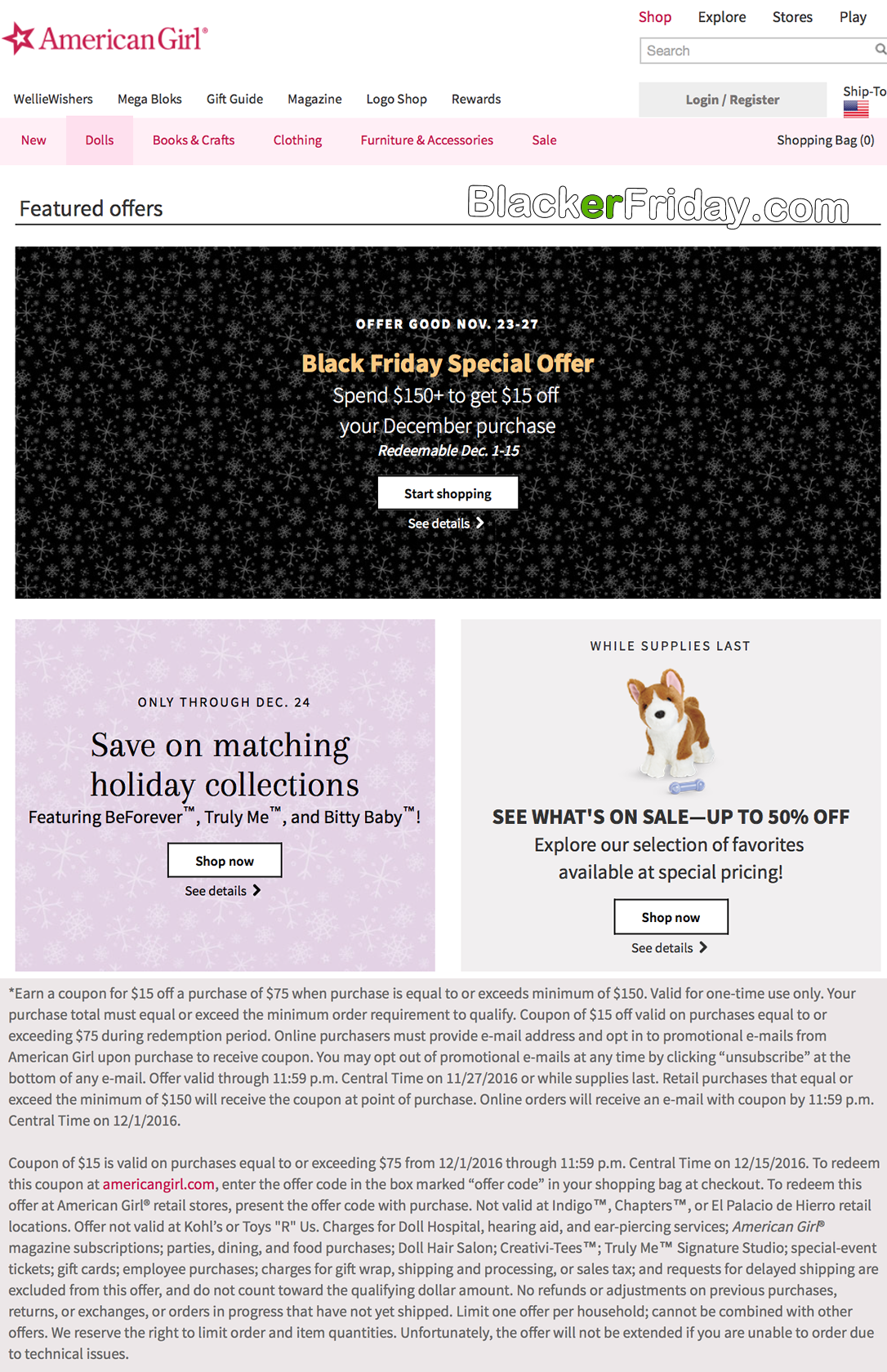This image captures a webpage from the American Girl website. The top section features a white background with a slightly tilted pink star containing a smaller white star inside, located in the top left corner. Beside the star is the text "American Girl."

To the right, there’s a white search bar with a gray border, labeled "search," accompanied by a search icon. Above the search bar, the word "Shop" is displayed in pink, followed by "Explore," "Stores," and "Play" in black text.

Beneath the "American Girl" logo, the navigation continues in black text: "Welly Wishers," "Mega Bloks," "Gift Guide Magazine," "Logo Shop," and "Rewards." 

To the right of the search bar, a small blue tab labeled "Login/Register" in black text can be seen. Below this, a white background features "Ship To" in black text next to an American flag icon.

The left section below the main navigation bar has a pink border with various category links in a darker pink: "New," "Dolls," "Books & Crafts," "Clothing," "Furniture & Accessories," and "Sell." Similarly, on the right side, "Shopping Bag (0)" is displayed.

Centered beneath this, a white section with black text features "Featured Offers." Adjacent, inside a white box with a black border, the text reads "BLACK," with the "ER" in green, followed by "Friday.com." There is a black line and a small white border beneath this.

The next section has a black background with white text and snowflake designs, stating "Offer good November 23rd through 27th." Beneath this, a yellow text declares "Black Friday Special Offer," followed by more details about the offer. A white tab labeled "Start Shopping" and a link to "See Details" are below.

To the left of this section, a pink background with white snowflake motifs announces an offer valid "Only through December 24th." To the right, another offer appears on a light blue background with the text "While Supplies Last" next to a plushie dog image. It invites visitors to "See what's on sale up to 50% off," with a "Shop Now" tab beneath.

The bottom section of the image has a light blue background filled with text — approximately seven lines of a paragraph, a small space, followed by about ten lines of additional information.